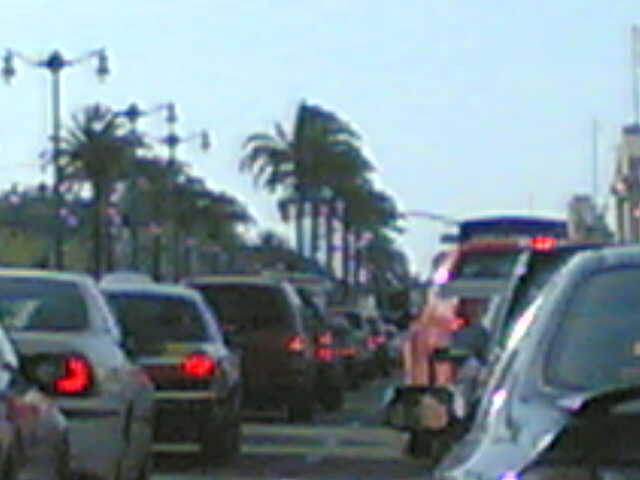This blurry daytime photo captures a standstill traffic jam on a highway, possibly located in California or Florida, indicated by the row of stately palm trees lining the road. The light blue sky stretches above, with street lights visible but unlit due to the daylight. Two lanes are completely stopped, their brake lights glowing in unison. On the right-hand side, the tops of a building are partially visible above the line of cars. In the foreground, the left side mirror of a car reveals the reflection of a woman, adding a human element to the scene of congestion.